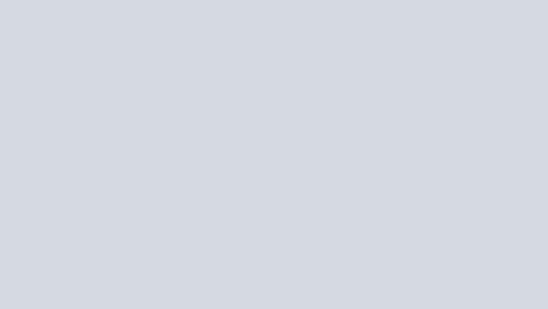This image features a completely blank rectangle set against a white backdrop. The rectangle itself is a light grey hue, slightly darker than the pure white surrounding it. There are absolutely no textual, visual, or graphical elements present within the grey rectangle—no discernible content or distinguishing features that can be analyzed or described. The stark simplicity of the image, devoid of image data or any differentiating marks, emphasizes the uniformity of its light grey color.